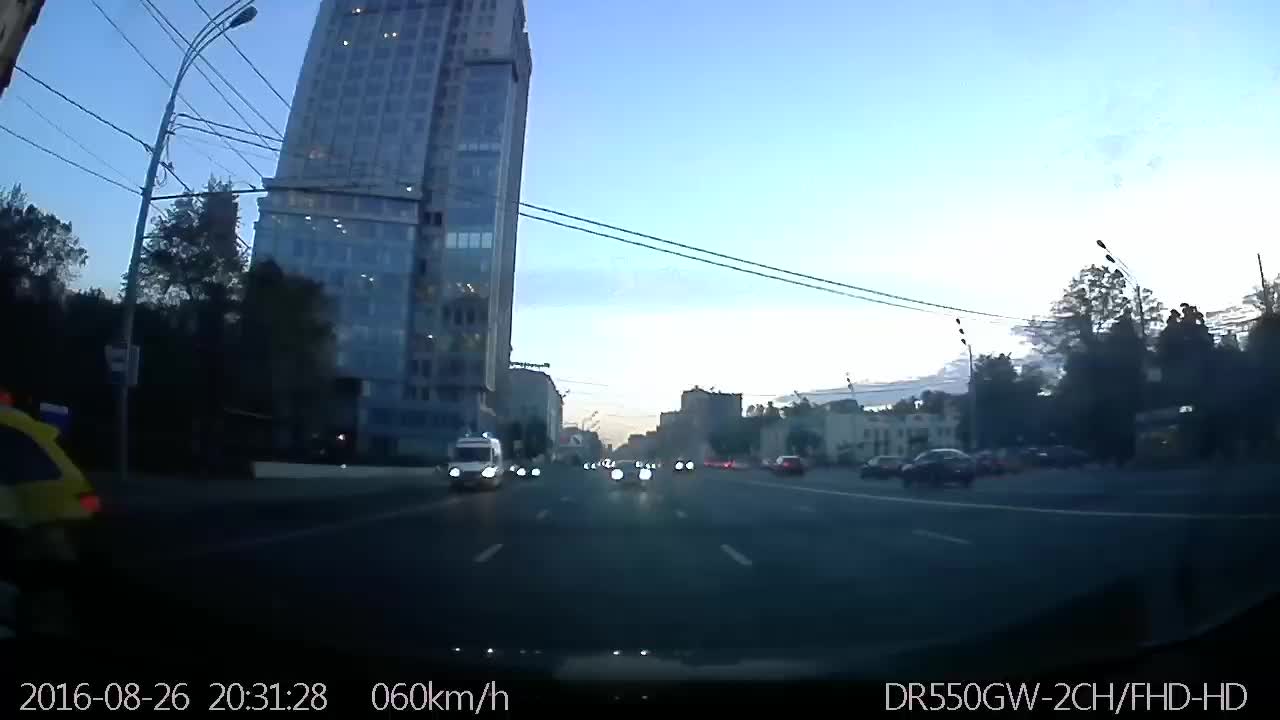This image appears to be a screenshot likely taken from a rear-facing dash cam mounted on a vehicle. The photograph captures a wide, three-lane asphalt road with clearly marked white dashes. Oncoming traffic is seen heading towards the camera, suggesting that the camera is situated at the back of the vehicle. The sun is low on the horizon, indicating either sunrise or sunset, casting a warm glow on the scene. A prominent skyscraper with numerous windows dominates the background, adding an urban touch to the setting. Additionally, a light pole with several electrical lines stretches across the top of the highway. The lower part of the image features data overlay, including a date and time stamp, providing contextual information about when the image was taken.